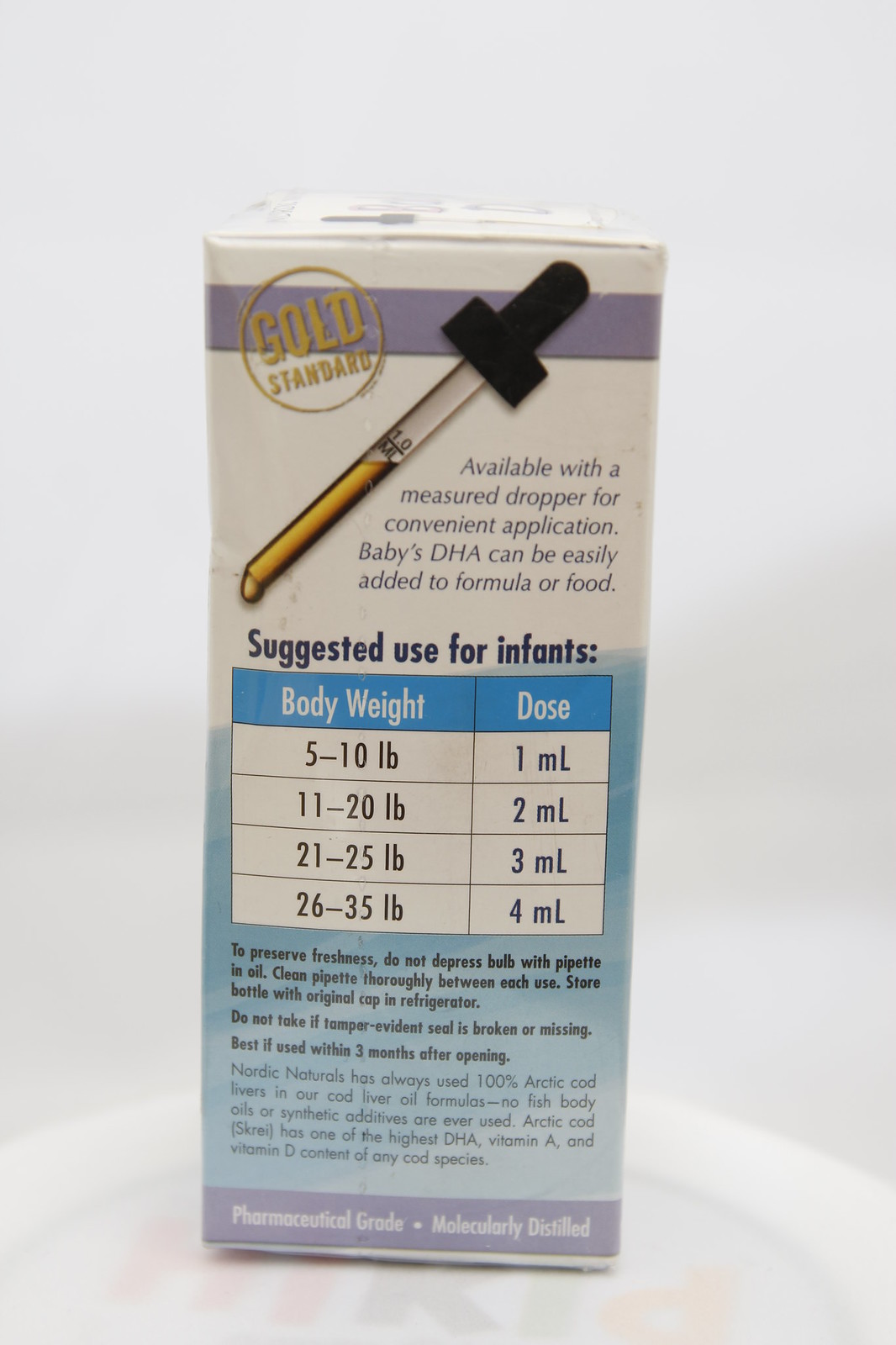This photograph displays the back of a tall, slender cardboard package positioned against a white backdrop that is not entirely pure, revealing some shading on the surface and background. The package is relatively small and primarily designed for baby DHA supplements. At the top, there is a prominent gold circle featuring bold capital letters that read "GOLD STANDARD." Adjacent to this is an icon depicting an eyedropper containing golden liquid. Below these visuals, there is text stating, "Available with a measured dropper for convenient application. Baby's DHA can be easily added to formula or food." Further down, the packaging provides guidance on dosage, detailing recommendations based on the weight of different infants.